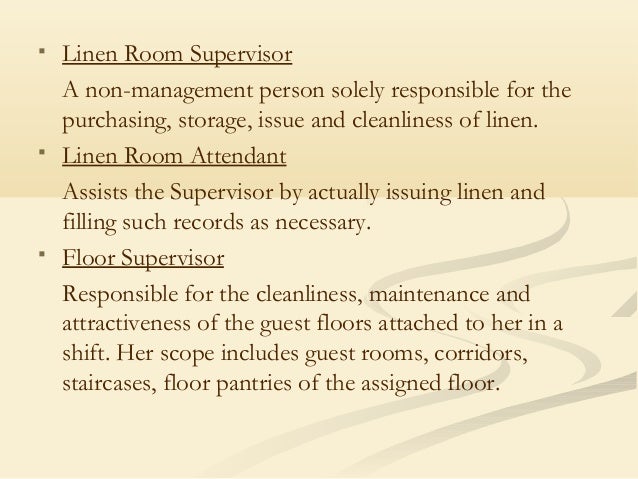This image is a detailed job description slide designed in a landscape orientation with a beige-ish tan and creamy background. The top third of the slide features a darker cream color, while the bottom two-thirds showcase a lighter cream color with a light gray swirl pattern on the right. The text is aligned to the left and appears in black, possibly brown, using a Times New Roman-like font. There are three square bullet points, each describing specific roles and responsibilities. 

The first bullet point is “Linen Room Supervisor,” described as a non-management person solely responsible for the purchasing, storage, issuing, and cleanliness of linen. The second bullet point, “Linen Room Attendant,” assists the supervisor with issuing linen and filling records as necessary. The final bullet point, “Floor Supervisor,” is responsible for the cleanliness, maintenance, and attractiveness of the assigned guest floors, including guest rooms, corridors, staircases, and floor pantries during her shift. The entire slide combines graphic design with typographic elements to convey the information clearly.